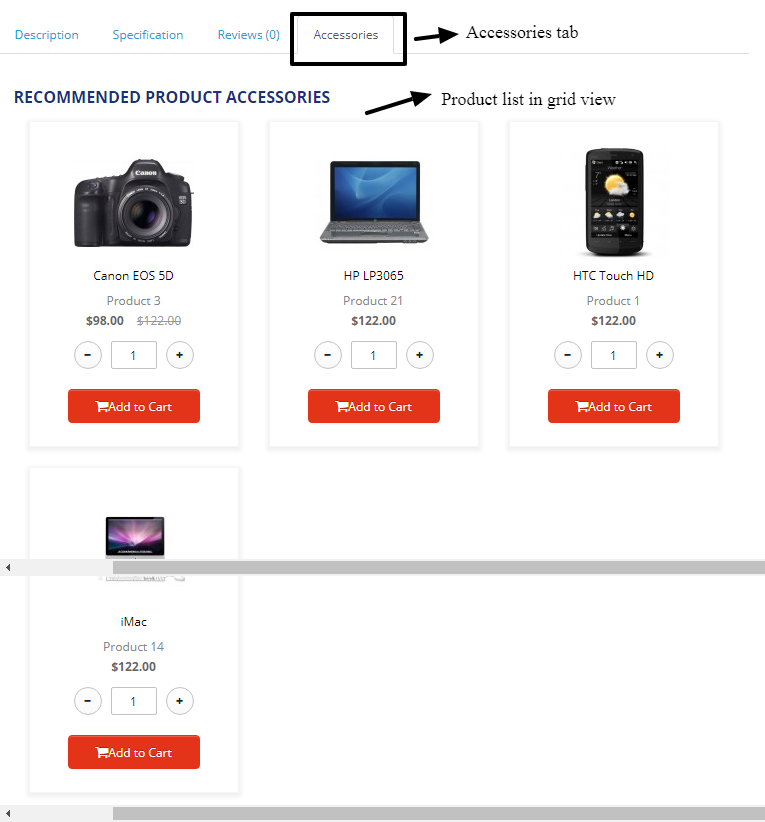This screenshot depicts a shopping page on a website with a clean, white background. At the top of the screen, several tabs are present, labeled from left to right as Description, Specification, Reviews, and Zero, all in blue text. The selected tab, Accessories, is highlighted in black text with a white tab around it, encased within a black box and indicated by an arrow with "Accessories tab" overlay.

In the main content area, a heading titled "RECOMMENDED PRODUCT ACCESSORIES" appears in all caps and blue text. Below this, four products are displayed, each enclosed in a vertical rectangle outlined with a light gray shadow and a white background. 

1. The first product is a black DSLR camera, labeled "Canon EOS 5D, Product 3." Its price is listed as $98, discounted from the crossed-out price of $122. The quantity is set to 1. Beneath the description, a red "Add to Cart" button is displayed, with "Add to Cart" written in white text alongside a white cart icon.

2. To the right, a laptop labeled "HP LP3065, Product 21" is priced at $122 with a quantity of 1. It also features a similar red "Add to Cart" button at the bottom.

3. Next, an older model touchscreen cell phone, labeled "HTC Touch HD, Product 1," is also priced at $122 and has a quantity of 1. It includes the standard "Add to Cart" button below.

4. The final product, located at the bottom-left, is a Mac computer with a keyboard and mouse, labeled "iMac, Product 14," priced at $122 with a quantity of 1, and includes the "Add to Cart" button as well.